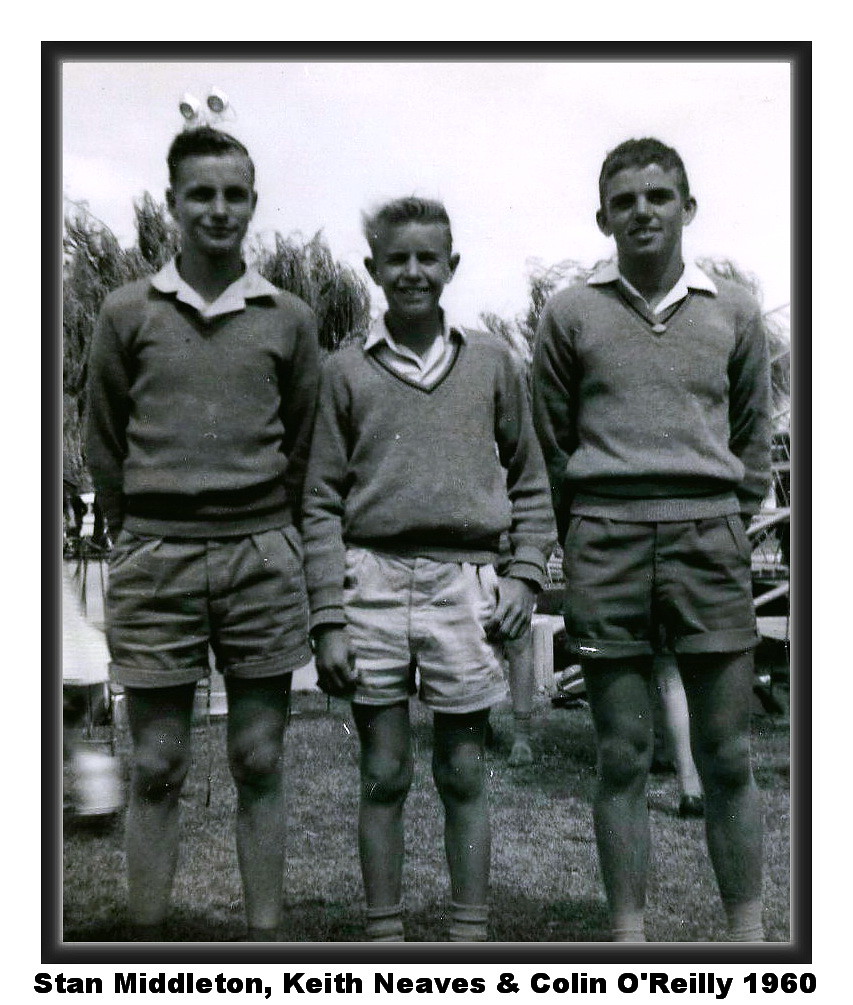This black-and-white image from 1960 features three young men, likely in their teenage years, standing outdoors in a grassy area. Labeled at the bottom as Stan Middleton, Keith Nieves, and Colin O'Reilly, the trio wears similar outfits consisting of shorts and collared shirts beneath sweaters. The two boys on either side are dressed in darker-colored shorts, while the one in the middle wears lighter shorts. All three have very short haircuts and are smiling. A peculiar detail includes what appear to be antennas on one of the boys' head, which could either be an accessory or an object in the background. The backdrop is a light, almost white sky, accompanied by visible trees and additional figures or legs suggesting adults nearby. A possible table and even a river can be seen in the distant background, adding to the image's nostalgic ambiance.